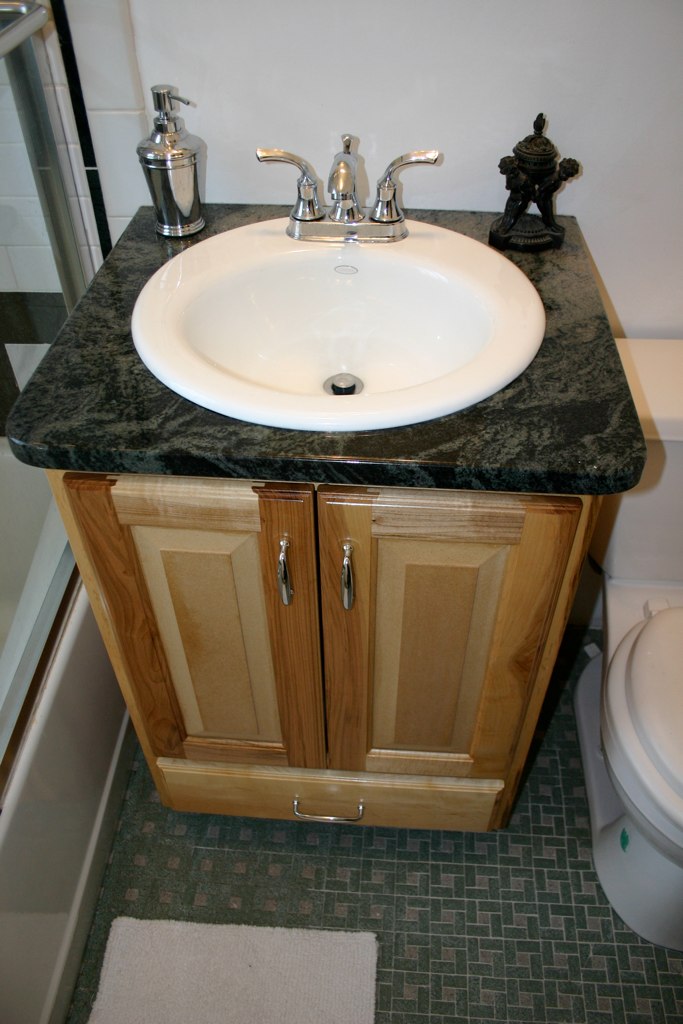This photograph captures a well-appointed bathroom with a single, oval-shaped white sink. Centrally located, the sink features a metal stopper at the bottom and is equipped with a single faucet that has separate pull handles for hot and cold water. Behind the faucet, there is a sink stopper lever. The sink is set into a sleek black granite countertop that showcases elegant gray swirls. 

To the right of the sink sits a decorative black ceramic figure with oriental design elements, adding a unique touch to the space. On the left side of the countertop, there is a shiny stainless steel soap dispenser, providing a modern, functional accent.

The sink and countertop are mounted on a wood cabinet with a rich walnut finish. This cabinet features brass handles and has a distinct square indention in its design. Below the two cabinet doors, there is a pull-out drawer with a matching brass handle.

The bathroom floor is tiled in a light and dark gray geometric pattern, enhancing the room's contemporary feel. A square cloth bath mat is placed on the floor, and you can see a tub situated next to the sink area, suggesting a clean and organized bathroom setup.